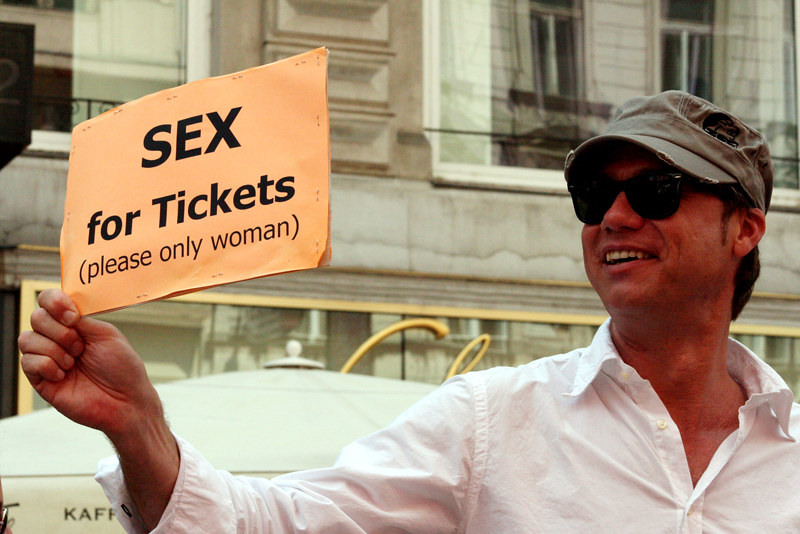In this outdoor image, a tanned Caucasian man is smiling as he holds up a light orange sign with bold, black text that reads "S-E-X for tickets" and beneath that, in smaller print, it says "(please only women)". He is wearing sunglasses, a white long-sleeve button-down shirt, and a gray cap. The man appears relaxed and cheerful. Behind him is a partly visible white and gray marble building with some gold edging and indistinct writing. Additionally, there’s a white tent or umbrella in the background, suggesting the photo was taken near an intersection, likely during an outdoor event.